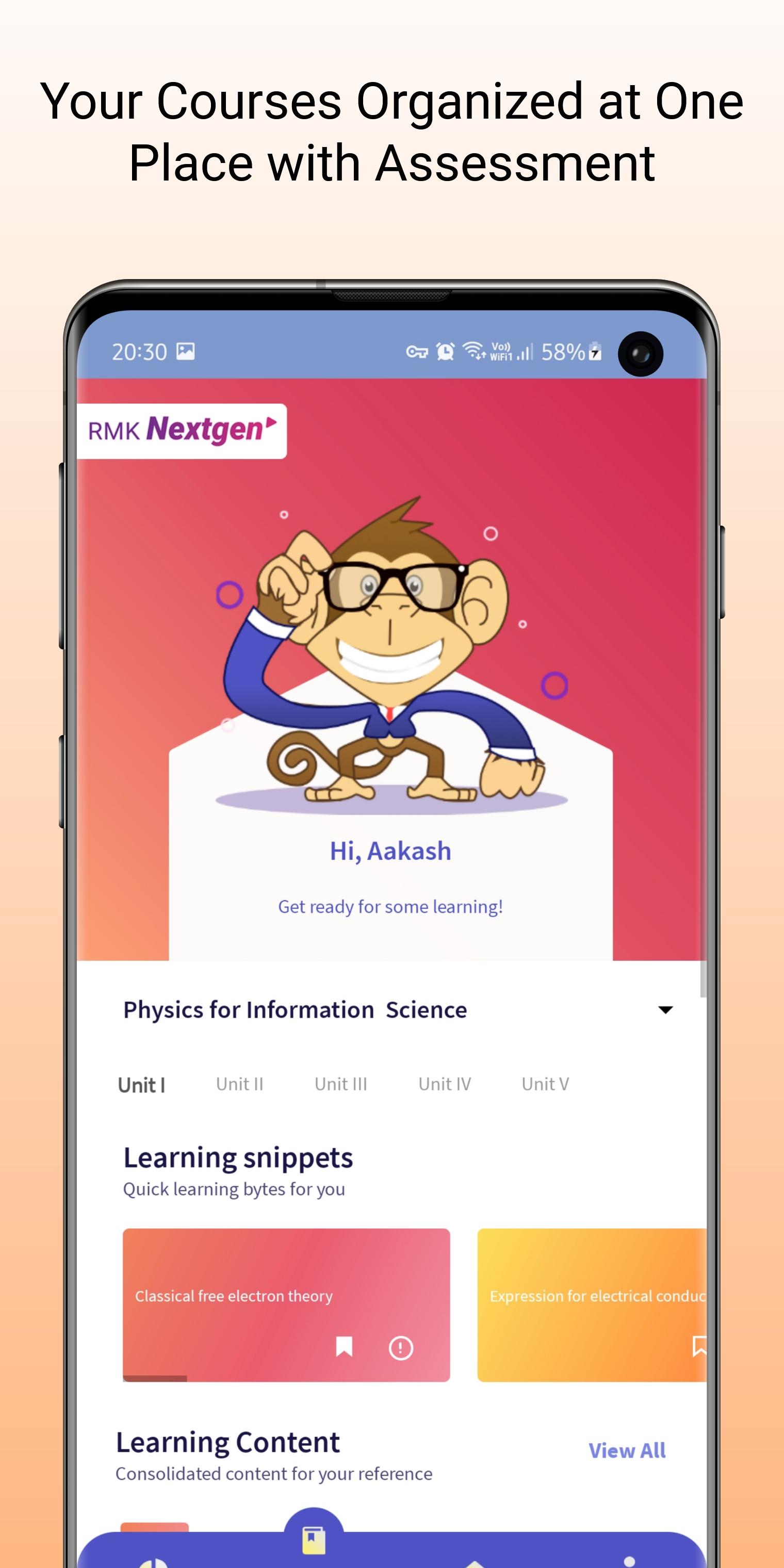The image is a screenshot of a cell phone interface displaying an educational app. At the top of the screen, on a peach-colored background, there is text in black that reads, "Your courses organized in one place with assessment." Below this header, the screen features a button labeled "RMK Next Gen," accompanied by a right-pointing arrow, indicating it is clickable.

Centered on the screen is a whimsical cartoon character: a monkey. The monkey wears black glasses, a blue suit coat, a white dress shirt, and a red tie. It is depicted sitting on an envelope while reaching up to adjust its glasses. Its tail is curved artistically at the end.

Beneath the monkey, bold text greets the user with, "Hi Akash, get ready for some learning." Following this welcome message, the screen lists a course titled, "Physics for Information Science." Each unit of the course is listed sequentially with Roman numerals: Unit I, Unit II, Unit III, Unit IV, and Unit V.

Further down, there is a section labeled, "Learning Snippets: Quick learning bites for you," featuring two clickable rectangles likely leading to additional content. The screen concludes with various learning materials available at the bottom.